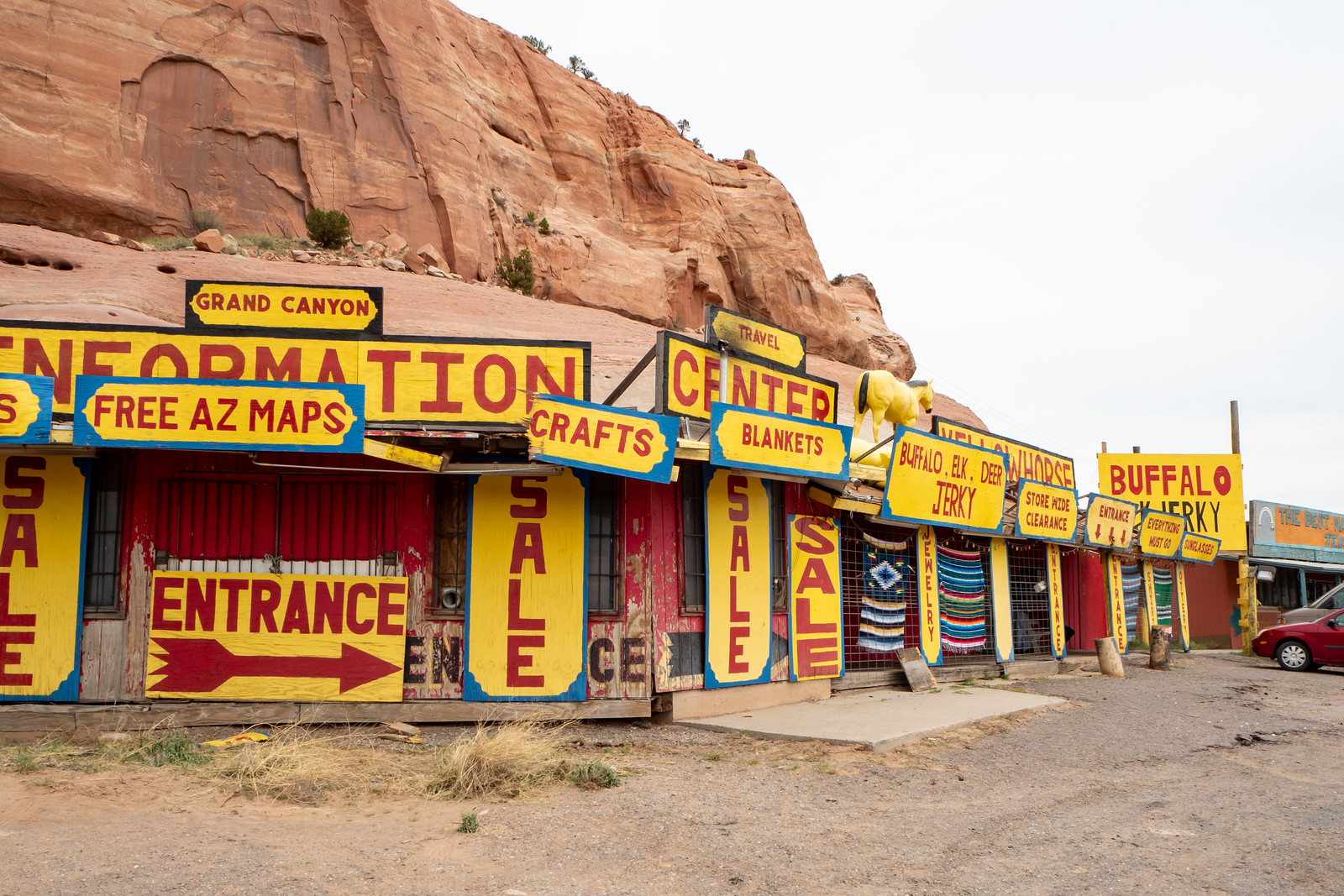The image depicts a quintessential roadside attraction, seemingly from a bygone era, nestled against a striking beige rock outcropping, reminiscent of the Grand Canyon's rugged landscape. This unique venue, possibly called "Yellow Horse," appears to be built directly into the rock, giving it an almost cavernous look. The ground in front of the storefronts is dirt, adding to the rustic charm of the setting.

A row of storefronts and entryways is adorned with a plethora of colorful, hand-painted signs in bright yellow with red fonts and blue borders, giving off a circus-like vibe. The signs, overlapping each other, advertise various offerings such as "Grand Canyon Information," "Free Arizona Maps," "Crafts," "Travel Center," "Blankets," "Buffalo Elk and Deer Jerky," "Storewide Clearance," and "Sunglasses," among others. The repetitive "Sale" signs emphasize the bustling, almost carnival-like ambiance of the place.

Adding to the scene's authenticity, there are traditional Native American rugs displayed, and atop one of the structures sits a small statue of a yellow horse. Parked cars to the right suggest visitors frequent this charming, offbeat stop, piquing the interest of travelers seeking a unique roadside experience.

An air of nostalgia pervades the photo, making it an intriguing snapshot of Americana, and its distinct characteristics mark it as the kind of peculiar yet fascinating spot you'd encounter while journeying along historic routes like Route 66 or near national treasures like the Grand Canyon.